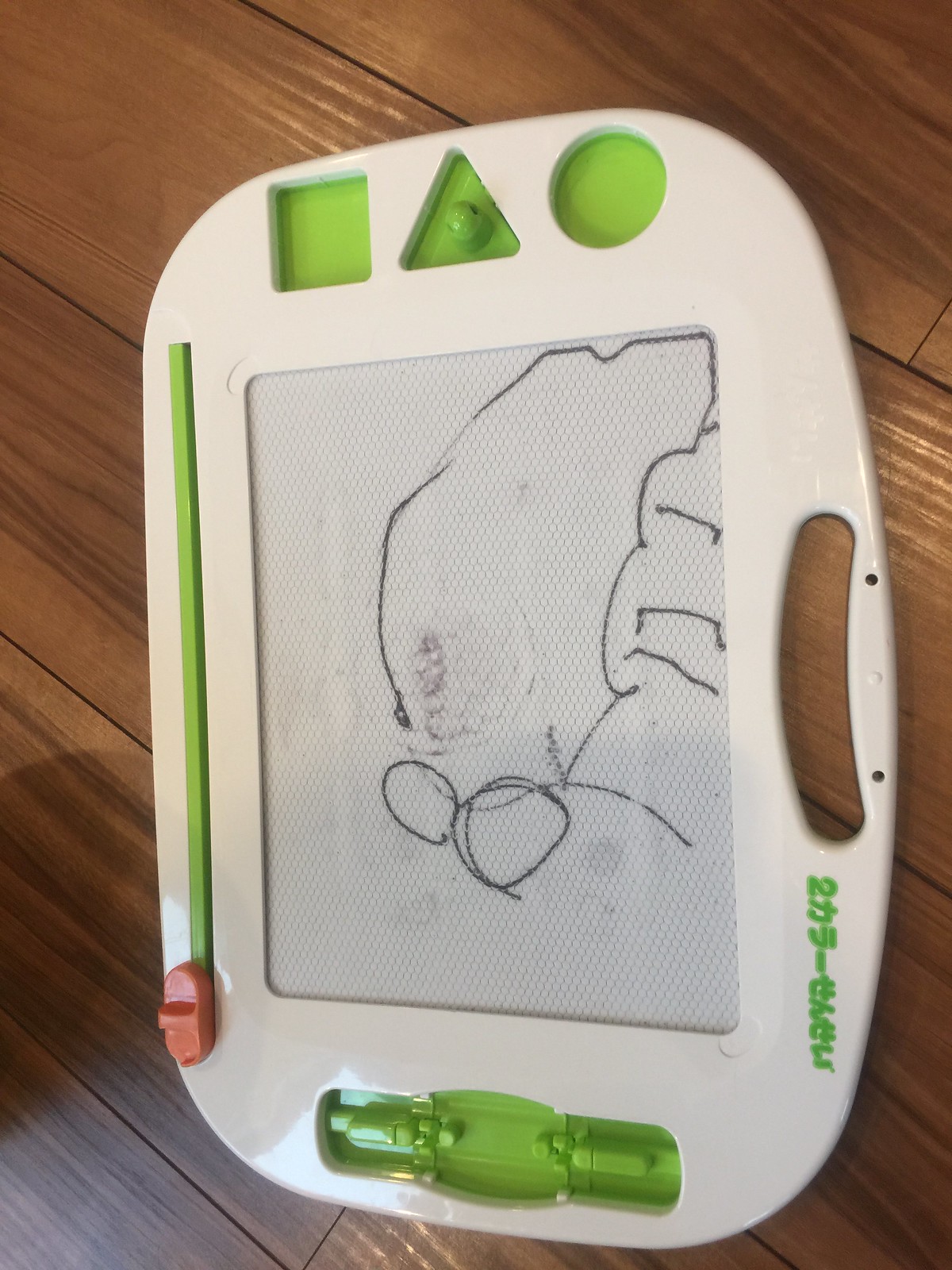This image features a child's toy called a Magnadoodle, characterized by a rounded but rectangular white plastic frame with light green accents. It is oriented vertically, showing the entire toy in what would typically be its portrait mode. The drawing surface is white with a textured appearance composed of small octagon shapes. At the top of the Magnadoodle, there are three green shapes: a square, a triangle with a magnetic stamp resting on it, and a circle. The pen holder, situated at the bottom, is light green and empty, indicating the pen is missing. On the left side of the toy, an orange slider allows for easy erasure of drawings. The Magnadoodle currently displays a child's drawing, featuring two large, bulging eyes, a body, and four stick-like legs, resembling an abstract animal or bug. Near the top handle, there is some Asian writing in green, possibly the logo of the manufacturer, though it is indecipherable. The entire toy sits on a medium wood slat floor.